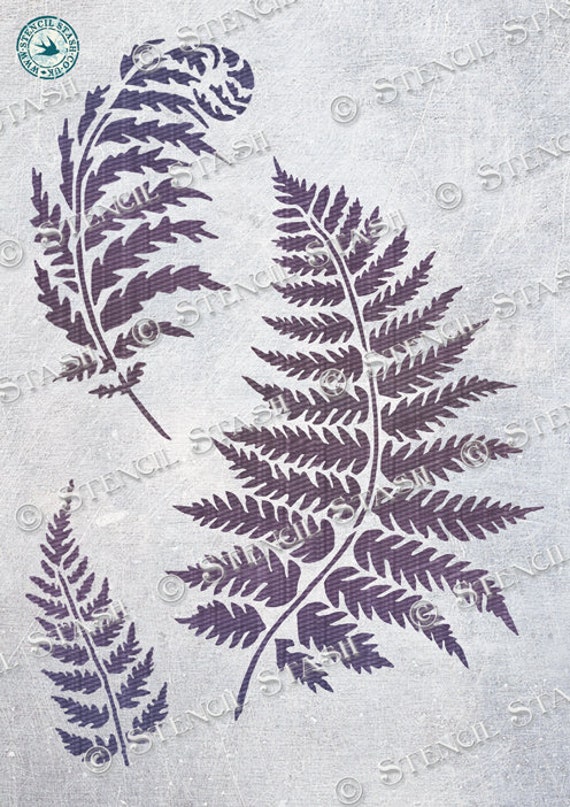This image features three distinct stencils positioned against a light gray-white background. In the center-right, there's a larger, detailed stencil resembling a stylized fern or a branch from a fir tree, characterized by a central twig and numerous spiky offshoots, much like a Christmas tree's branches. To the top left above it, there's a similar but slightly different design: the leaves are more rounded, less pointy, and the overall shape curls upward like a feather. A smaller version of the central stencil is present in the bottom left. All stencils appear executed in a dark, almost black color. Repeatedly overlaying the image is a watermark that reads "Stencil Stash copyright." Additionally, in the top left corner, there is a circular green logo containing the website "www.stencilstash.co.uk" and a small black bird in the center. This collection suggests these intricate and textured plant designs were created for stencil use and then meticulously scanned or photographed.